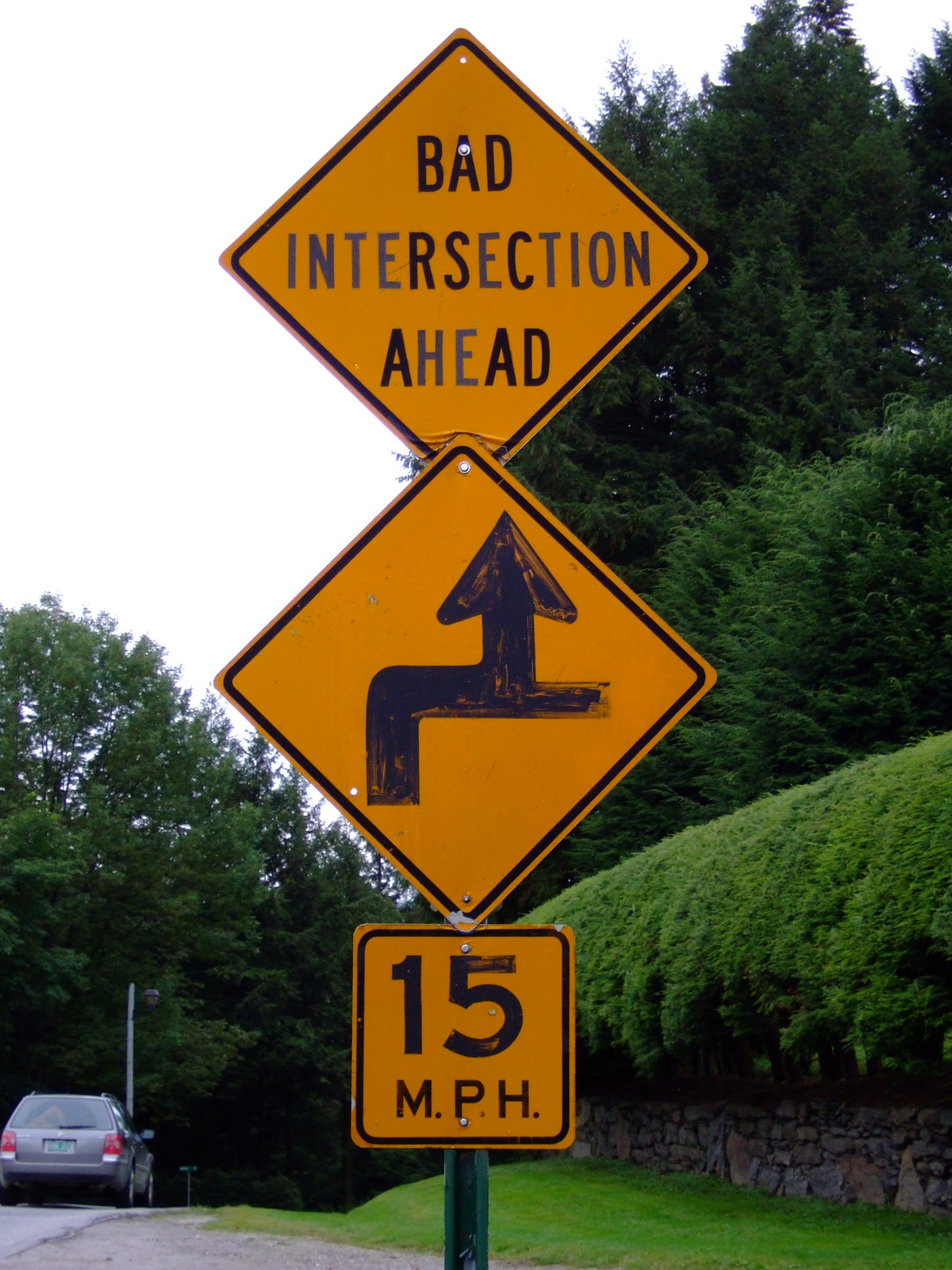This image features a prominent road sign mounted on a green metal pole, deeply embedded into the ground. The pole supports three distinct signs. At the top is a yellow diamond sign with black lettering that reads "Bad Intersection Ahead." Below it is another yellow diamond-shaped sign depicting a diagram of a complicated roadway. The diagram illustrates a route that ascends, sharply curves to the right, and then branches into two directions, either continuing forward or veering right. The bottom sign is a small yellow square indicating a speed limit of 15 miles per hour.

In the background to the left, there's intricately landscaped bush hedging with a stone border, complemented by a well-maintained grassy area. Tall poplar trees can also be seen along the left side of the road, creating an enveloping green canopy. Additionally, a car, which appears to be a minivan, is discernible on the road, adding to the scene's dynamic nature.